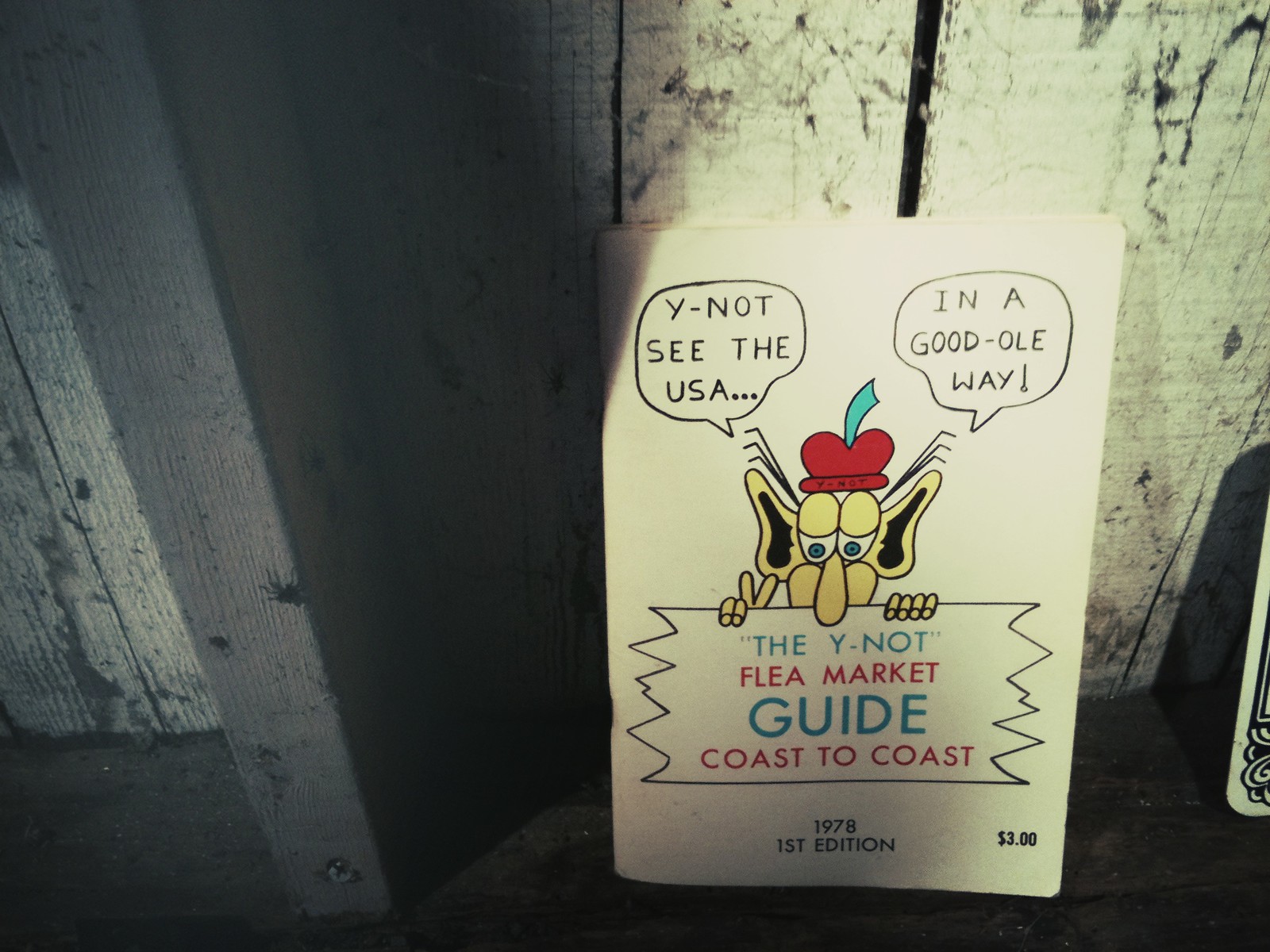The photograph depicts an aging wooden building with vertical white planks showing signs of wear, cobwebs, and dirt, creating brown spots and darkened areas. Natural light focuses on a distinctive sign positioned toward the bottom-right center of the image. The sign features a cartoon character with large, blue egg-shaped eyes, a long oval nose, and prominent egg-shaped cheeks. This character has exaggerated elephant-like ears, a red hat with a blue feather, sparse strands of hair, and exhibits a playful expression while holding up two fingers in a peace sign with the right hand. The sign itself, appearing like a squiggly cutout, includes two speech bubbles: "Why not see the U.S.A.?" and "In a good ole way." It advertises "The Why Not? Flea Market Guide, Coast to Coast," identified as the first edition from 1978 and priced at three dollars. This quirky advertisement leans against part of a weathered door frame, enhancing the rustic charm of the setting.